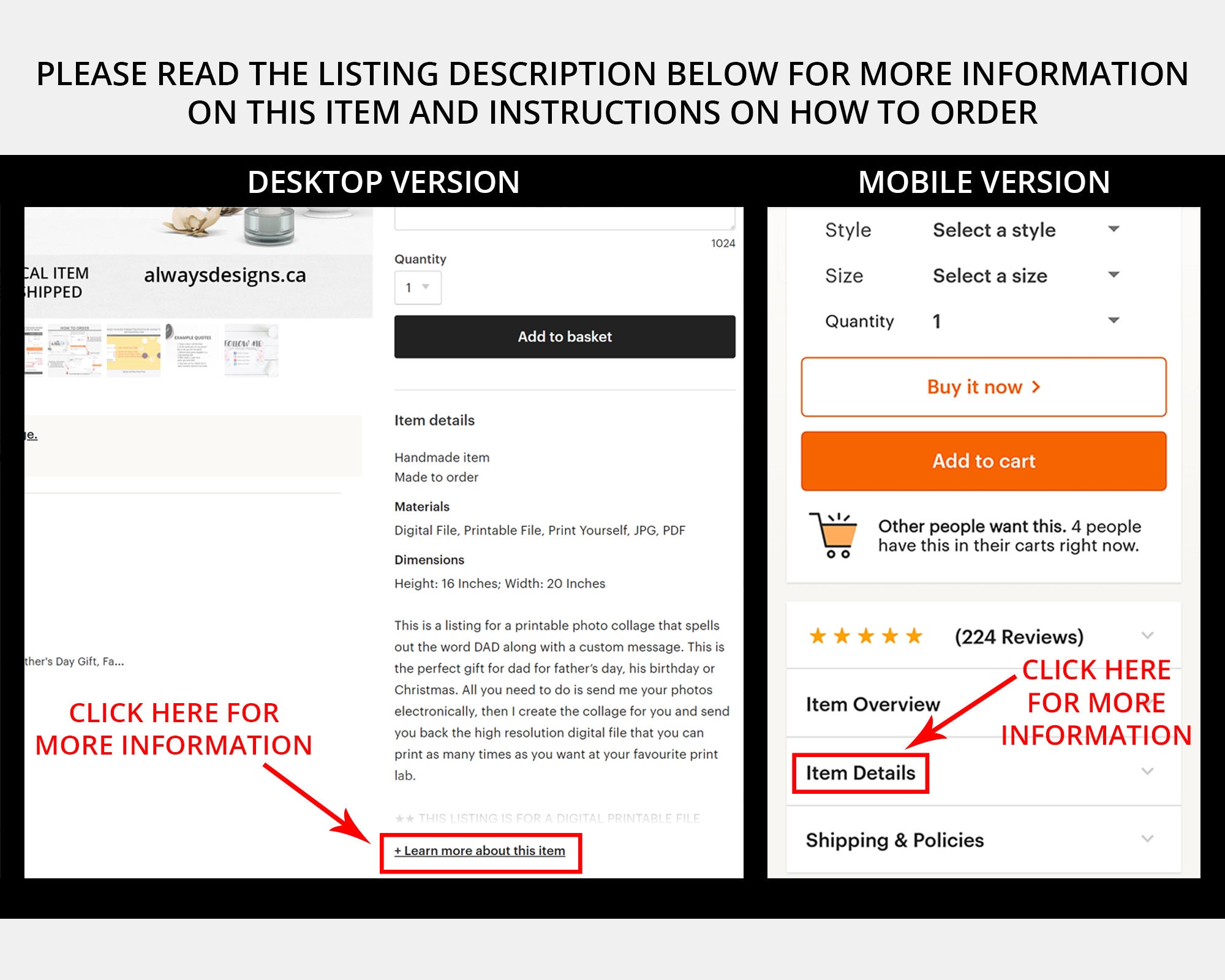The image features a gray bar at the top with black, all-capitalized text spanning two lines, which reads: "PLEASE READ THE LISTING DESCRIPTION BELOW FOR MORE INFORMATION ON THE ITEM. INSTRUCTIONS ON HOW TO ORDER."

Beneath this bar, the image is divided into two sections with a black background. The left section represents the desktop version, depicting a screenshot with a red arrow pointing to a link labeled "Learn More About This Item" at the bottom. The right section illustrates the mobile version, showcasing a screenshot with a red arrow pointing to an "Item Details" option, accompanied by the text "Click Here for More Information" in red font.